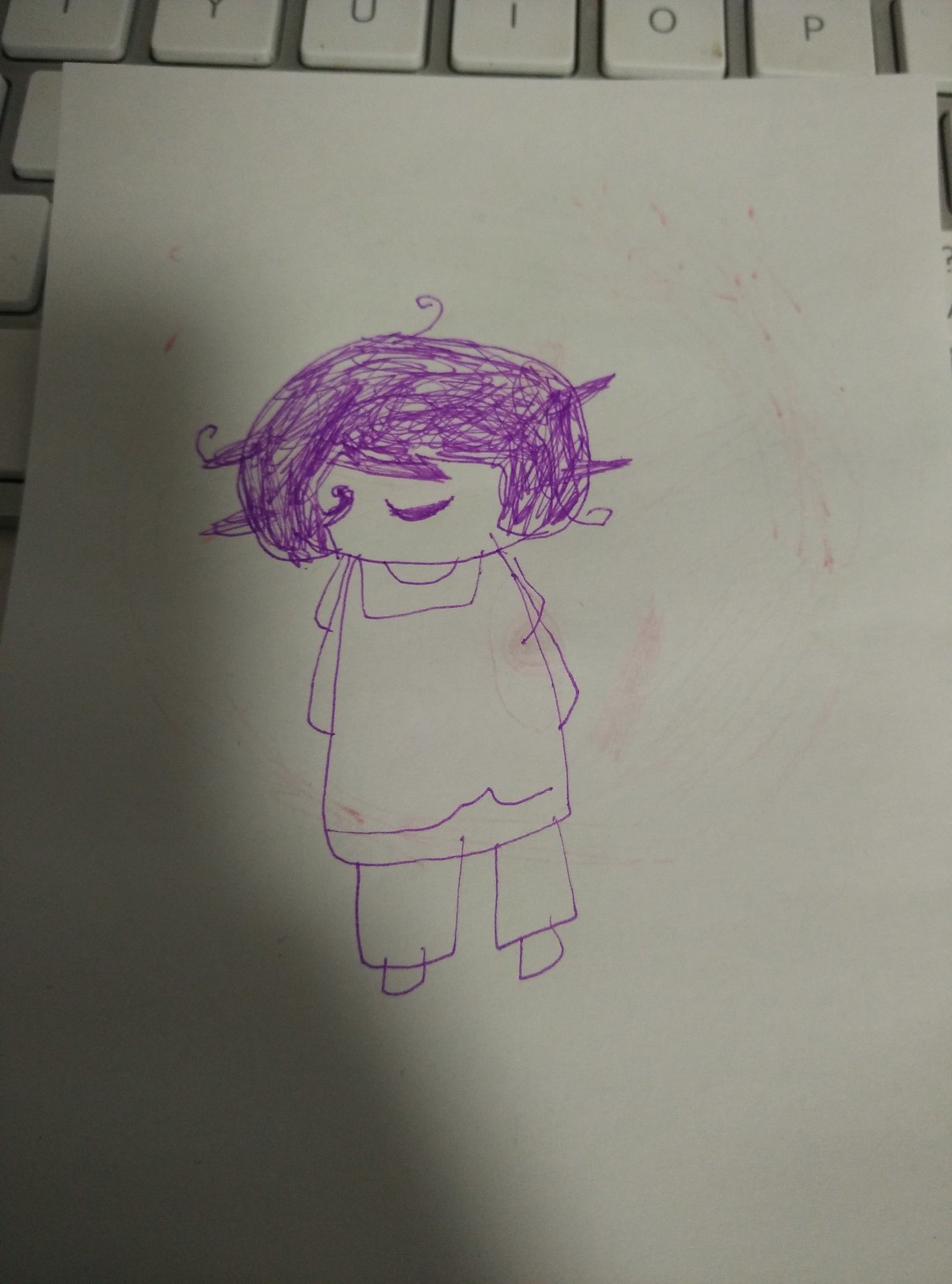This color photograph showcases a simple line drawing, likely created by a child, placed on a keyboard. The lighting in the image is poor, casting a greyish tint over elements that are probably white. The photograph reveals a piece of white paper positioned atop the keys, with the U, I, O, and P keys clearly visible along the top left edge.

At the center of the image, drawn in purple ink, is a whimsical representation of a woman. Her curly hair cascades over her eyes, and a cheerful smile adorns her face. Her elongated torso is complemented by small, round arms positioned behind her body. She appears to be dressed in a uniquely styled outfit: a square-shaped upper garment next to a long, rimmed tunic that flares slightly at the hem. Her attire extends to white trousers, with her feet represented by two small square shapes.

Adding to the composition, a dark shadow descends from the top towards the middle bottom edge on the left side of the photo. The overall effect highlights the charming simplicity of the child's drawing against the everyday backdrop of a computer keyboard.